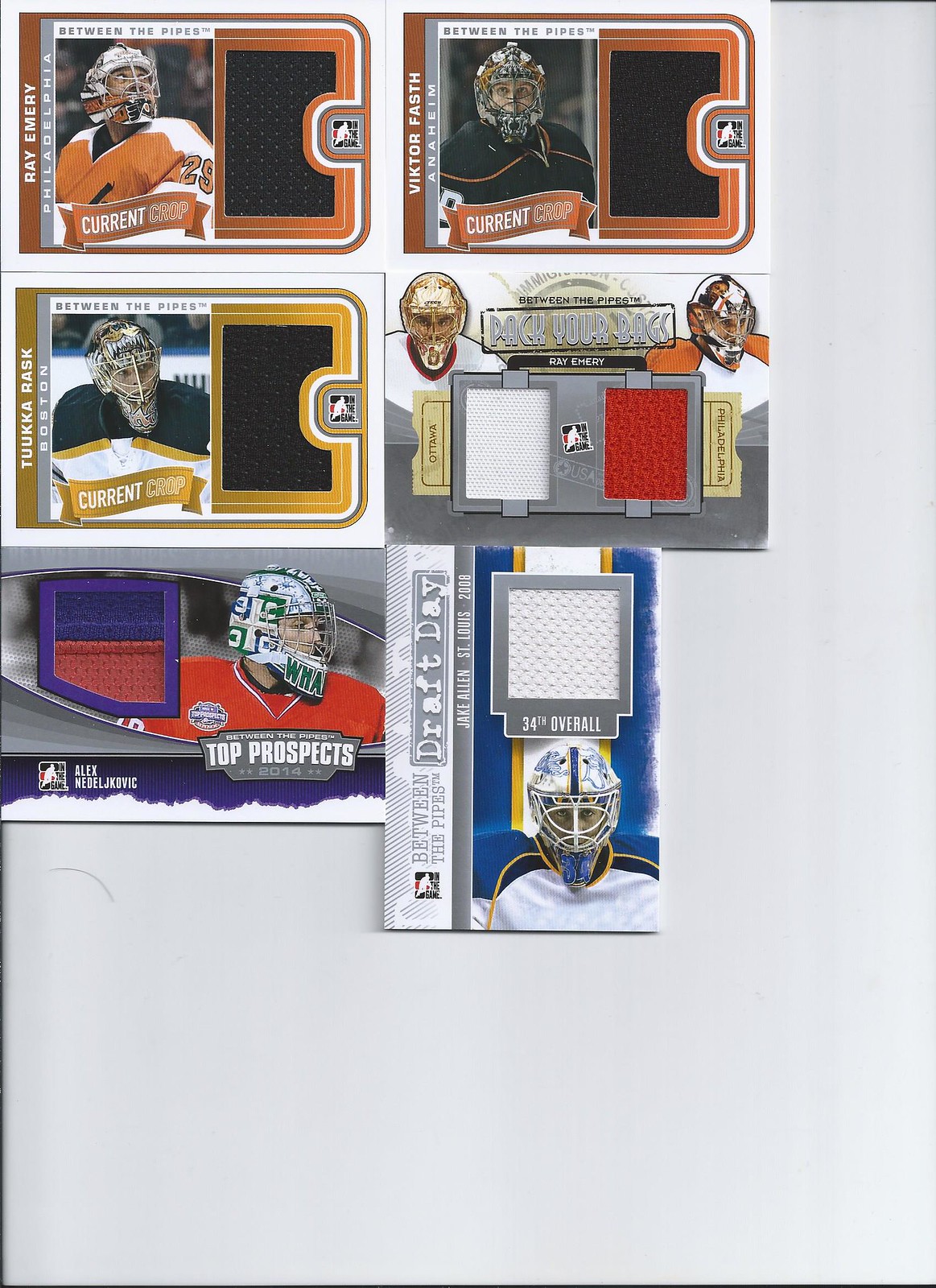The image displays six hockey trading cards arrayed against a white background. The top row features two cards with a white and copper design: the first card, on the left, showcases Ray Emery in uniform with the caption "Current Champ." Next to it on the right is a similar card for Victor Fasth, also labeled "Current Champ." The middle row's first card has a white background with a gold border and presents Tuka Rask in uniform, including his helmet, with the player's name written along the side in white. Adjacent to this, the second card in the row has a white background showing two players in uniform, though the text between them is not readable. The bottom row includes a card with a gray background featuring a player in a red uniform, captioned "Top Prospects," while the final card displays a background of blue, white, and gold, titled "Draft Day, 34th overall."